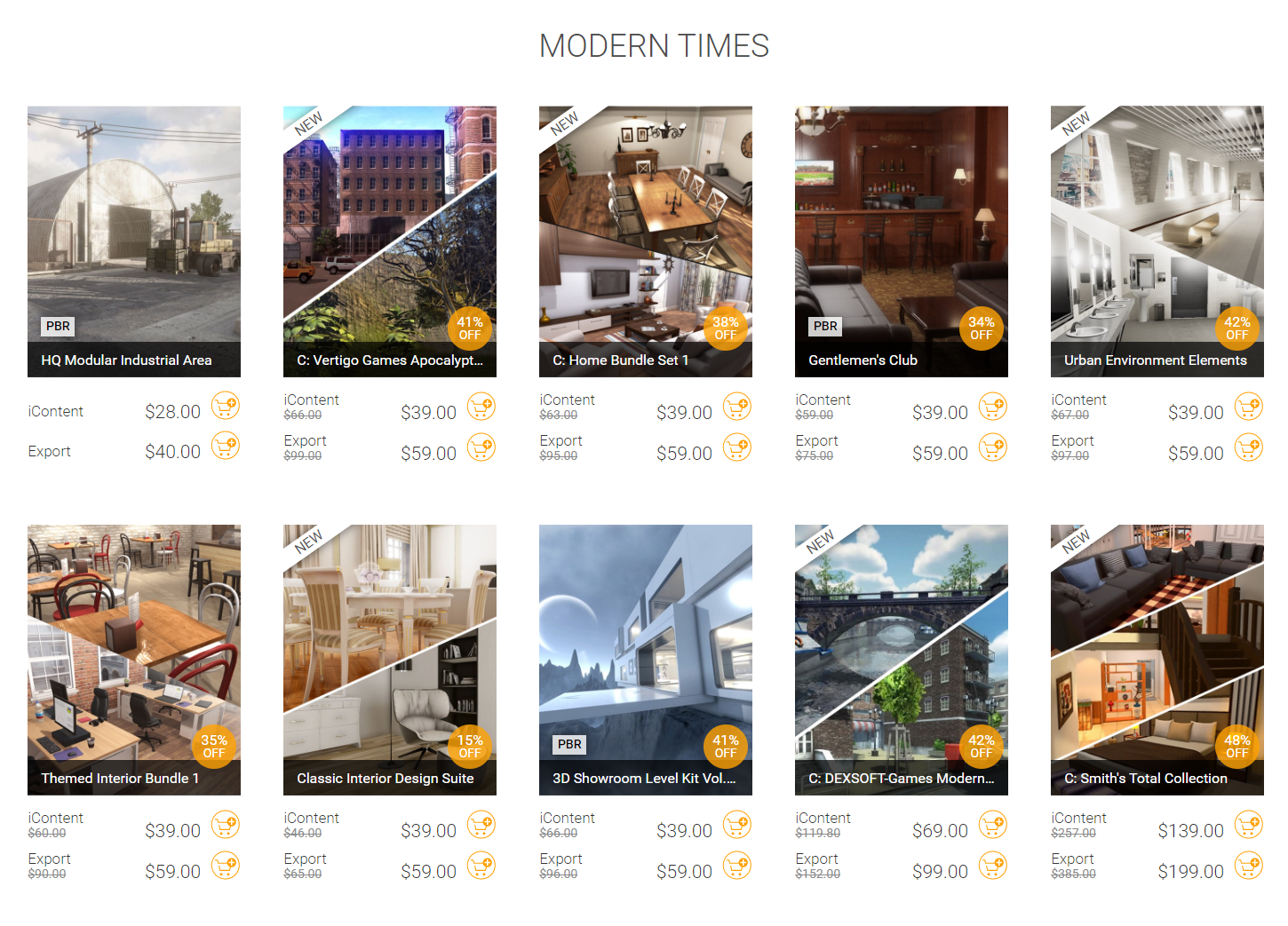**Image Caption:**

At the top center of the image, "MODERN TIMES" is prominently displayed in capitalized dark gray lettering. The layout features several elements towards the left, including images of a circular building, a utility pole, and a tractor-like vehicle positioned towards the center-right.

The bottom footer of the image is black with white text that reads "HQ, Modular Industrial Area." Towards the top left of this footer, there is a small white rectangular icon with the capitalized black text "PBR." Below this icon in gray text, it says "eye contact." To the right, the text "$28" is displayed next to a shopping cart symbol bordered by a circular orange frame. Further to the right, it says "export" in black, followed by the text "$40" accompanied by another circular bordered orange cart icon.

The second section of the image showcases a diagonal slashed view. On one side, there is a corporate cityscape with various vehicles, numerous brown buildings, and a blue sky. A white ribbon at the top of this section reads "new." The opposite side reveals a nature scene with a tree and a bush in the bottom left corner. The footer for this section is black with white text that reads "C:\\Vertigo Games, Apocalypse..." (which is partially cut off). In the upper right of the footer, there is a circular transparent orange icon with white text stating "41% off." Beneath this in gray text, it says "eye contact." Adjacent to this, there is a slashed price of "$66," reduced to "$39," followed by the same circular bordered orange cart icon seen previously.